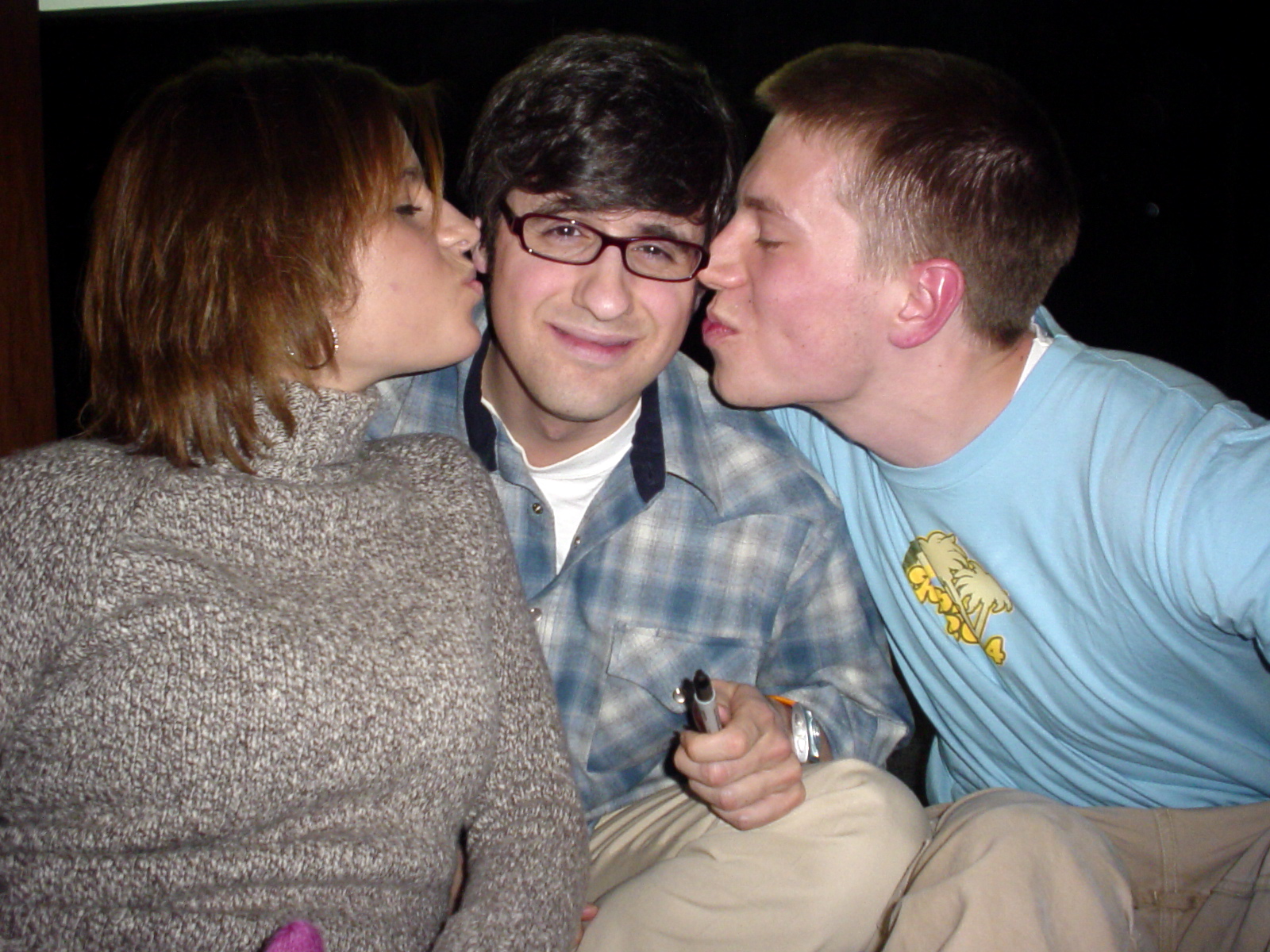In this photo against a dark background, we see three friends engaging in a playful moment. At the center is a young man with short, dark brown hair, parted and swept to the left. He wears dark brown oval-framed glasses and sports a smile while holding a pen in his left hand. His attire consists of a blue plaid jacket over a white t-shirt and beige khaki pants, along with a watch with an orange strap on his left wrist. Flanking him on either side are a young woman and another young man, both seeming to lean in for a kiss on his cheeks. The woman on the left has short brown hair, adorned with silver earrings, and wears a gray turtleneck, her eyes gently closed in anticipation of the kiss. The young man on the right has light brown hair and wears a light baby blue t-shirt with some indeterminate design, along with tan cargo pants. The playful, affectionate scene captures a fun and intimate moment among the trio, set against an indiscernible dark background.